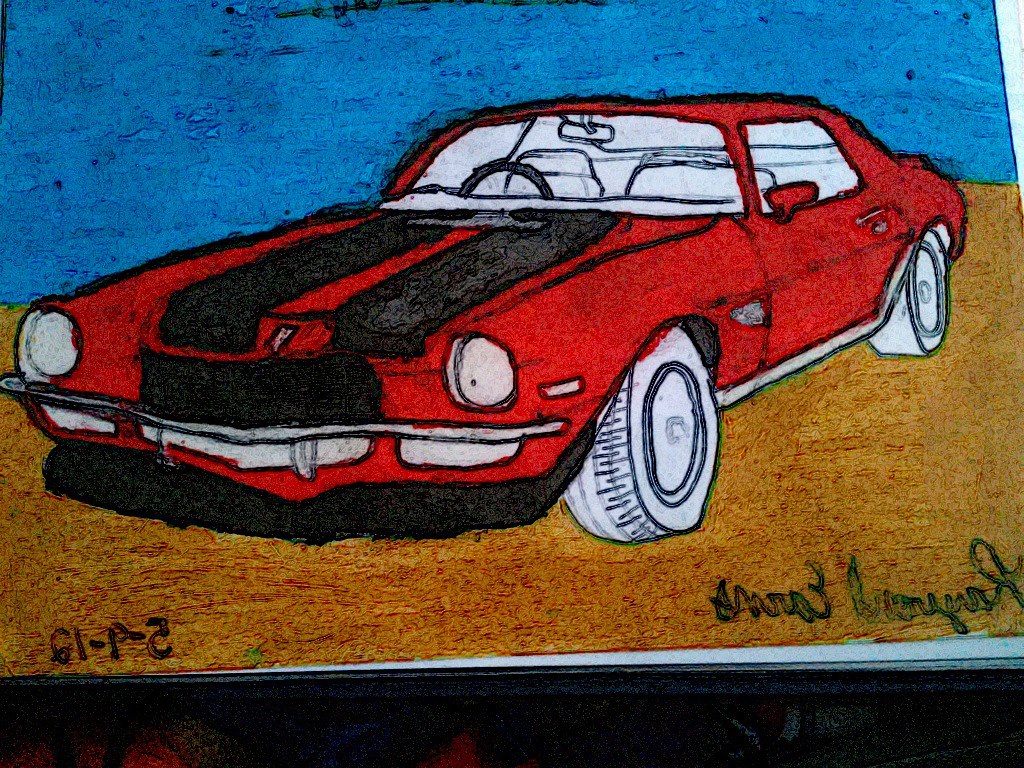This detailed, hand-drawn sketch features a classic, vintage sports car depicted from a front-three-quarter perspective. The vehicle, draped in an eye-catching red tone, boasts two bold, black racing stripes that run the length of its hood. Exhibiting a wide body, the car's design elements suggest influences from iconic models such as a Ford Mustang or a Chevrolet Chevelle, but the exact make remains unclear. The car's front presents a pair of prominent white headlights, flanking a shiny chrome bumper that exudes retro charm. The sleek two-door frame hints at a possible two-seater configuration, though the interior details remain ambiguous. A serene blue sky forms the background, contrasting with the brown-toned ground below, setting the car in an earthy, natural environment. The artwork, which appears to be rendered in watercolor, possibly markers, showcases the artist's dedication to detail and color harmony. Additionally, the drawing is signed, though the signature appears reversed, making it undecipherable. A backward date suggests the piece was completed in May 2012.